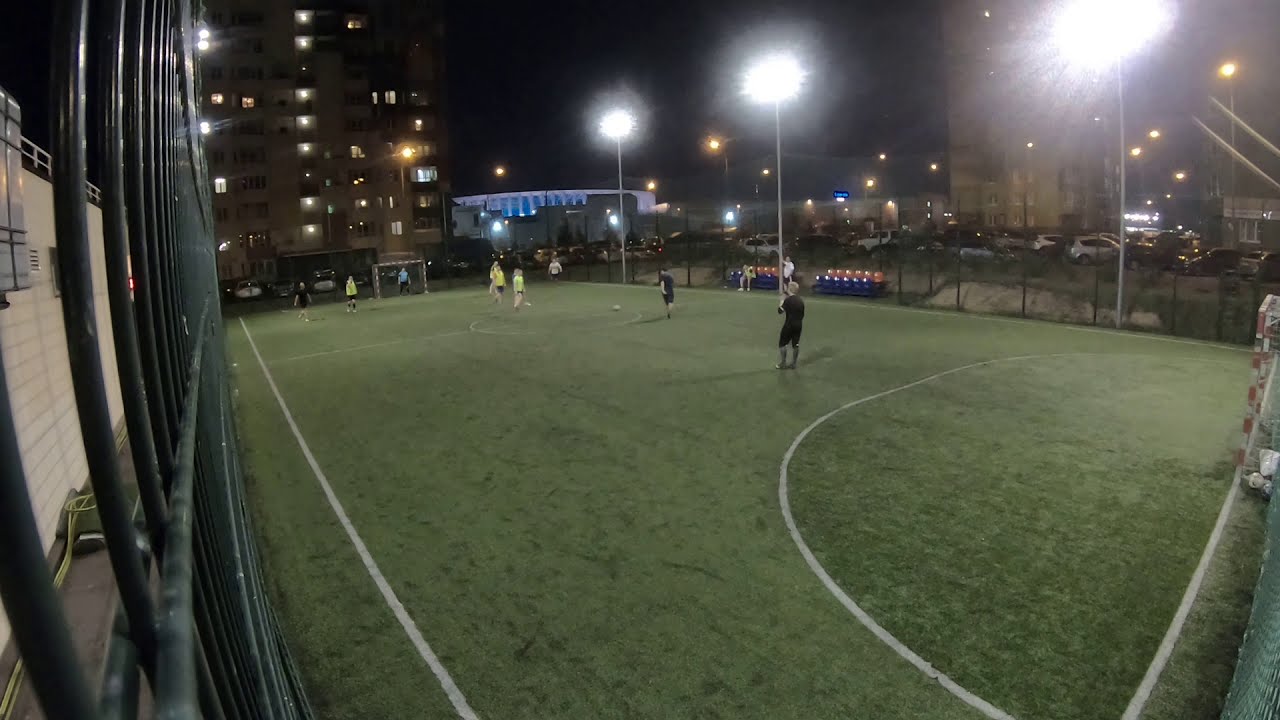This wide rectangular image captures a night scene of a small soccer field taken from the perspective of a corner. The field features green turf with white painted lines. The longer side of the field extends towards the left of the image, while the shorter side stretches diagonally to the right. On the left side, a tall black fence runs alongside the field, terminating at a white tile wall. At the opposite end, a gate leads to a parking lot filled with several cars. Tall floodlights illuminate the scene from the top of the image, casting bright white light over the field.

In the foreground, a three-on-three soccer game is underway. The players are divided into two teams — one in yellow and the other in black uniforms. Though their individual characteristics are not discernible due to the distance from the camera, the game appears casual, possibly just a practice session or a friendly match.

Surrounding the field, there are various tall buildings that could be apartments or office spaces. Additional amber street lights are visible in the background, further emphasizing the nighttime setting. The image is devoid of fans, but clearly shows the two goalposts at either end of the field.